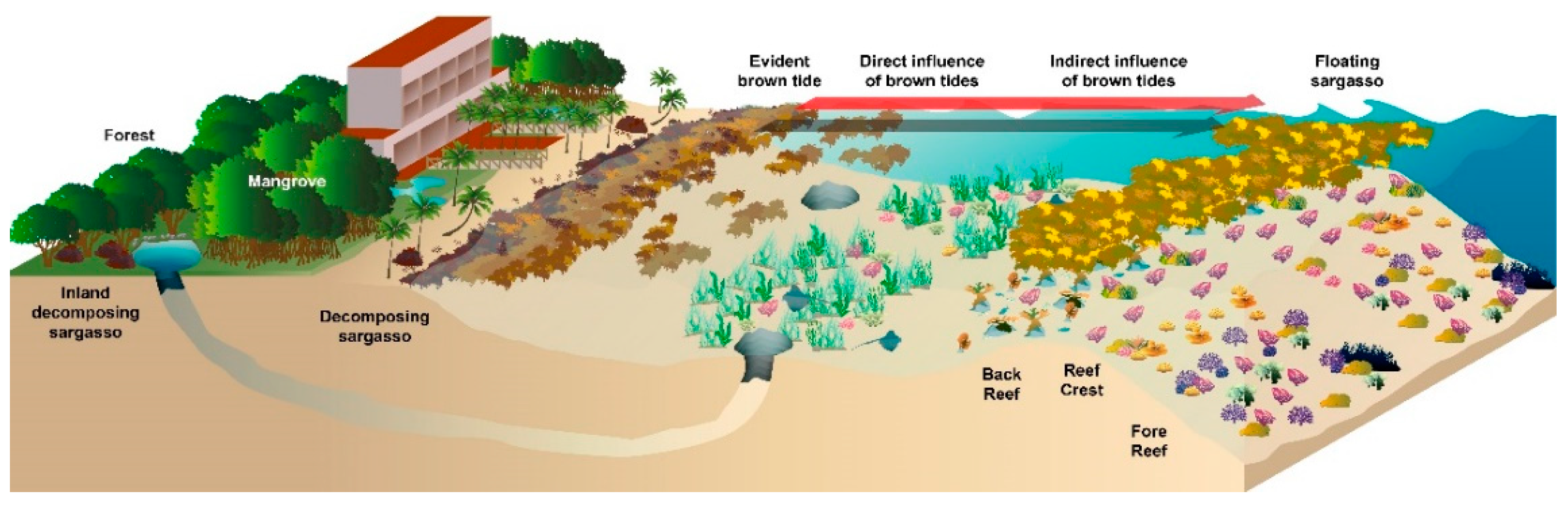This is a detailed animated illustration of a coastal area, emphasizing the interplay between different environmental zones and the impact of tides on coral reefs. The image is colored and labeled from left to right, featuring a two-story hotel surrounded by trees, facing out onto a body of water. The scene includes a beach area with distinct zones: a forest transitioning into mangroves, an inland pool labeled as decomposing sargasso, and patches of decomposing sargasso on the beach itself. The ocean is segmented into areas showing various stages of brown tide influence—evident brown tide, direct influence of brown tides, and indirect influence of brown tides—accompanied by floating sargasso. The diagram then illustrates the three distinct zones of the coral reef: the back reef, the reef crest, and the fore reef. This illustration effectively demonstrates how the forest, mangroves, and decomposing sargasso influence the tidal conditions and subsequently affect the health and state of the coral reefs.